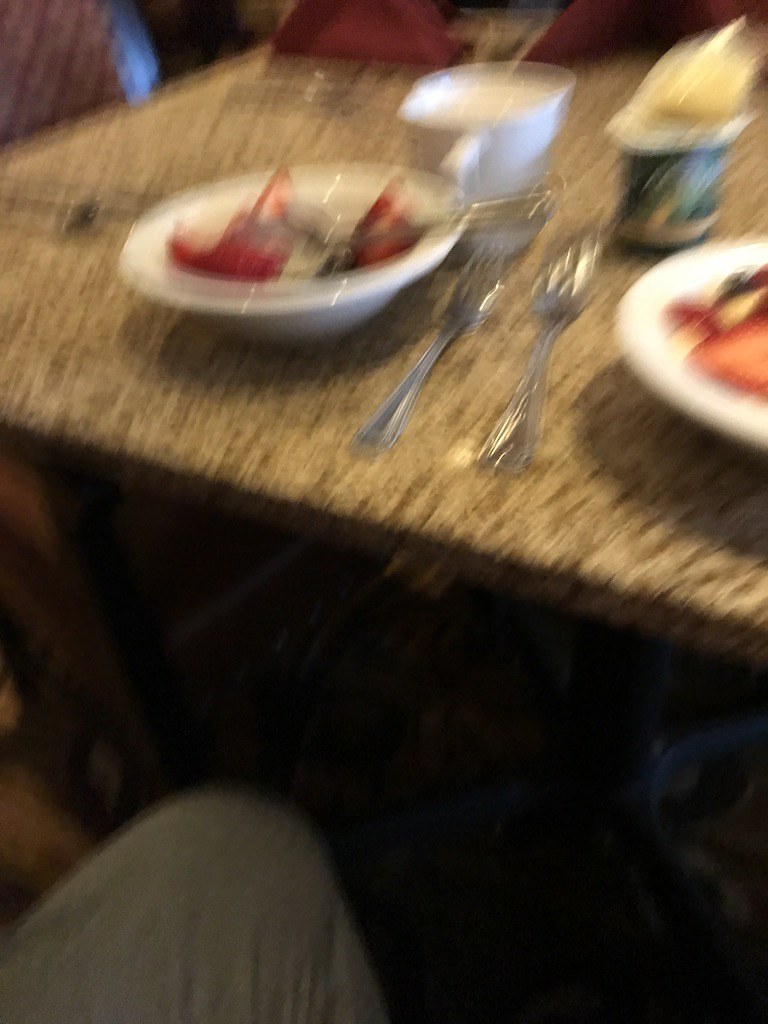A slightly blurry photograph captures a lively meal at a stone-textured tabletop, where a person's knee is visible, hinting at their seated position. The table features two white ceramic bowls filled with yogurt and garnished with sliced red strawberries. Beside the bowls, there are forks meticulously placed, ready for use. A white ceramic coffee cup stands prominently, adding to the breakfast ambiance. An open container of Activia yogurt with a green label is also present, indicating the source of the yogurt in the bowls.